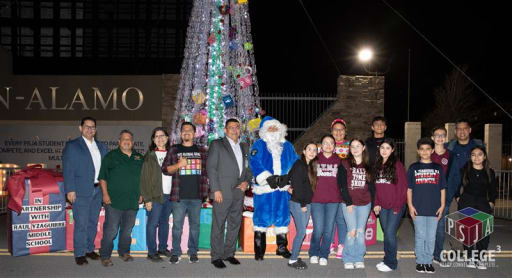This image captures a festive Christmas scene in a downtown city square, possibly during a charity event or school gathering. The central focus is on Santa Claus, who is uniquely dressed in a blue costume with white fur trim and black boots. Surrounding him are groups of students and adults. To Santa's left stands a man in a gray suit followed by four adults, likely in their 20s or 30s, with the last individual also dressed in a blue suit. On Santa's right, four children and teenagers stand in the front row, with boys donning blue t-shirts and jeans and girls wearing red hoodies. Behind them, four adults are aligned, with everyone facing the camera.

Directly behind this group is a shimmering Christmas tree fountain adorned with silver and green decorations, including hanging ornaments. A large wrapped gift in blue paper with a red bow sits to the left of the man in the gray suit. The package includes a message indicating a partnership with a middle school. On the left side of the image, a sign reads something-dash-Alamo, hinting at a possible school or location name. The bottom corners of the photo contain blurred text, with the right corner clearly stating "PSJA College." The color palette includes shades of blue, burgundy, red, green, white, tan, and beige, enhancing the holiday atmosphere.